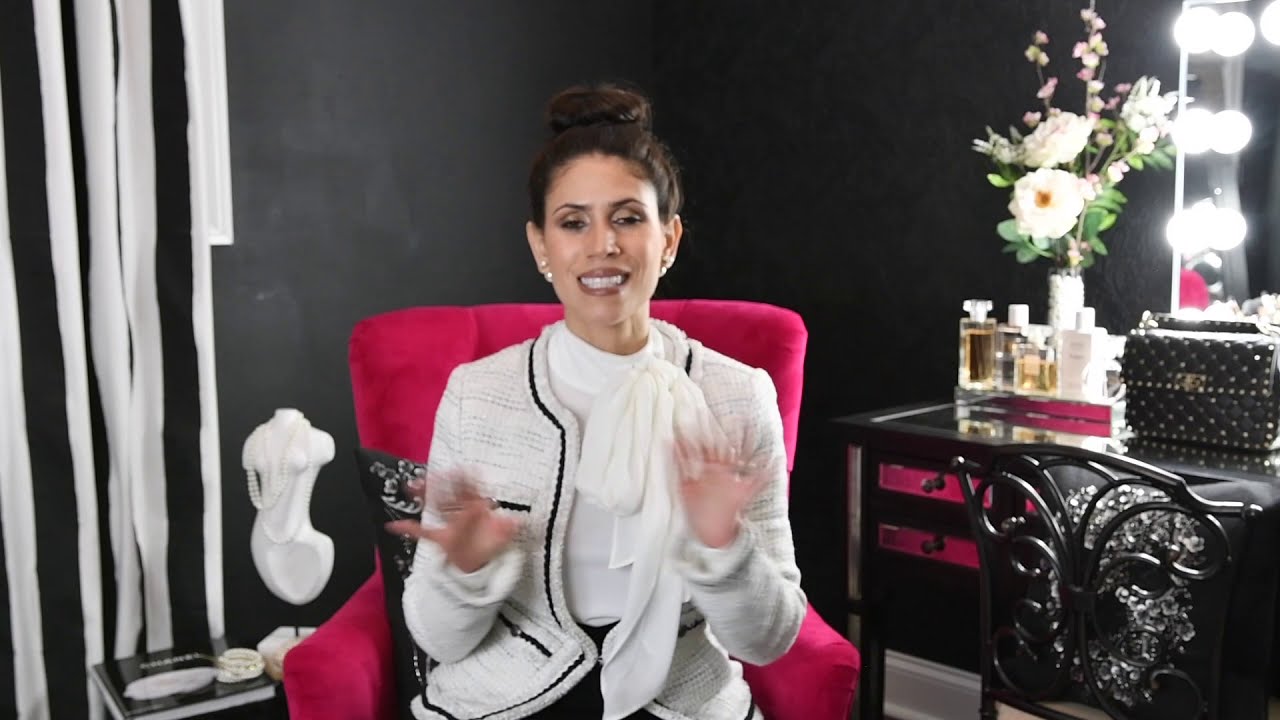In this detailed and vibrant image, a woman is captured mid-conversation, her hands raised in motion, creating a blur. She sits comfortably in a red velvet chair layered with a black pillow, dressed in a white sweater and a jacket with white and dark colored lines, her hair neatly styled in a bun. The background setting suggests a dressing room with a black wall adorned on the left side by a long white and black striped curtain, possibly outlining a window behind it. White ribbons are also seen hanging down from the wall on the left side.

To her right, a classic makeup mirror with light bulbs lining its edges is mounted on the wall, casting a soft glow over the scene. Below the mirror is a brown wooden makeup table with a glass top and two pink-handled drawers. On the table sits a brown box and an array of care products, including what appears to be bottles of perfume, lotions, and creams. Additionally, there's a small vase holding three white flowers, taller pink flowers, and a collection of leaves, alongside a black chair with an intricate design that gleams under the mirror’s light.

A statue, difficult to identify, stands on the table to the woman's left, adding an artistic element to the scene. A book rests on the same table, contributing a touch of intellectual allure. White ribbons on the left side of the wall add an accent of purity against the dark background, creating a striking contrast. The woman, smiling broadly with a full view of her teeth, appears engaged and lively, embodying a warm and dynamic presence amidst the detailed and thoughtfully arranged surroundings.